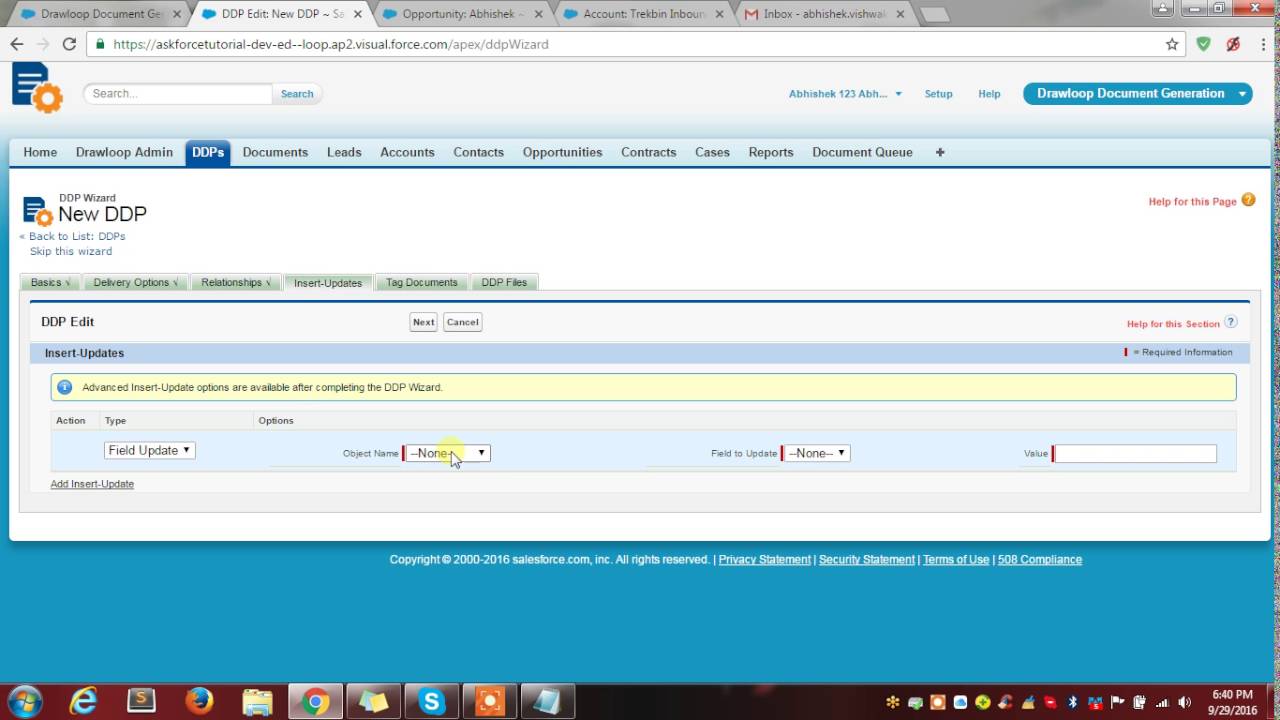A detailed caption: 

Displayed on the monitor are several open tabs on a web-based platform, showing a total of five active tabs. The primary tab showcases a CRM (Customer Relationship Management) interface labeled "New DPP." The interface consists of a blue-themed layout featuring a graphic element resembling a piece of paper, a gear icon, and a search bar situated prominently. Below the search bar, which contains the terms "Home, Drop Stop, DTP Documents, Leads, Accounts, Contacts, Opportunities, Contracts, Cases, Reports, Documents," is a blue button labeled "Drop Stop Document Generation."

The interface provides options for creating, editing, and updating various contact details and organizational data. Just beneath this section, there is a large bar, likely serving as a dynamic contact sheet where users can input and update the information of individuals they are communicating with, providing a comprehensive tool for managing ongoing communications and documentation.